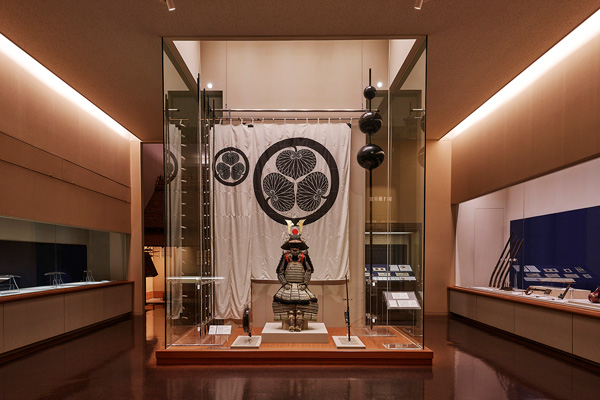This image captures an interior view of a sleek, modern museum room characterized by wood paneling that extends from the shiny wood floor up to the ceiling. The room, long and narrow, features glass display cases on either side, each with recessed lighting above, likely enhancing the observation of historical artifacts housed within. These cases are set into recesses and have shades that come down over long rectangular windows. Central to the image is a prominent glass display case resting on a wooden base; it extends nearly to the floor and showcases what appears to be a historical uniform, perhaps of Asian origin, complete with detailed elements such as boots and a skirt-like lower half that suggests armor, alongside other items like linens or blankets adorned with black circles and fan-like designs. The background reveals more of the museum’s space, indicated by a hanging tapestry with a circular design featuring spade shapes, and another figurine positioned on a desk. The overall ambiance is one of understated simplicity, directing the viewer's focus predominantly on the displayed artifacts.